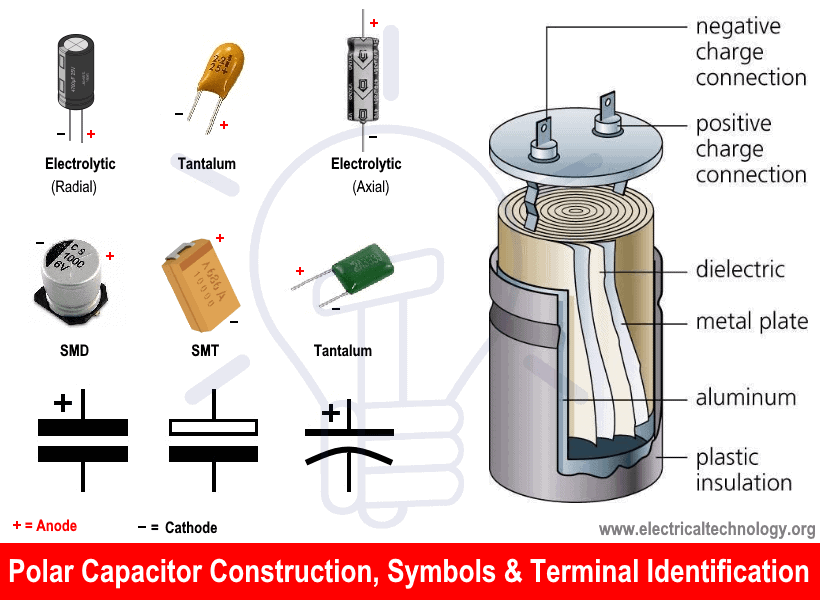The image, presented by www.electricaltechnology.org, depicts various polar capacitor construction symbols and terminal identifications against a white background with a red rectangular footer. Detailed annotations explain the internals of capacitors, highlighting the negative and positive charge connections, dielectric materials, metal plates, aluminum components, and plastic insulation. It features different capacitor types such as electrolytic, radial, tantalum, axial, SMD, and SMT, each marked with symbols. The symbols include black structures with plus signs, indicating anodes, and corresponding captions marking cathodes with minus signs. Additionally, a silver-colored disc atop a beige cylinder, enclosed by a silver exterior, is shown to illustrate capacitor components. The image is comprehensive, guiding viewers through electrical terminologies and parts with clear labels like anode (+) and cathode (-).